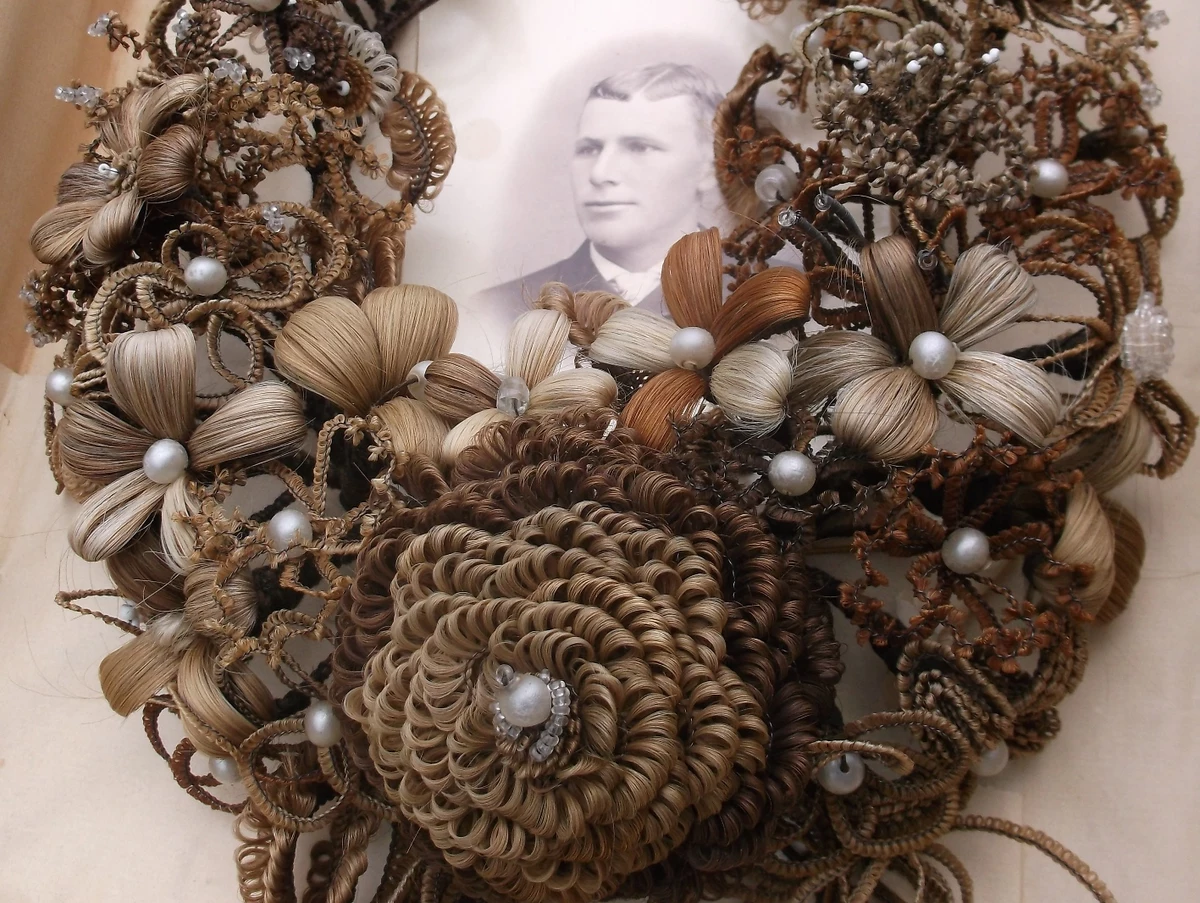This photograph features a black and white, oval-framed headshot of a Caucasian man, who has very short hair and is dressed in a black coat with a white shirt and tie. The portrait is set against a large white border and encased in a bronze-colored frame. This frame is adorned with an intricate, oval-shaped wreath made up of various thread flowers and pearls, giving it a delicate and ornate appearance reminiscent of a statement piece of jewelry. The wreath is primarily in shades of browns, tans, and oranges, embodying a vintage aesthetic. The top section of the wreath is unfortunately cut off at the edge of the photograph. This entire arrangement is placed on what seems to be a cardboard surface, likely for protection. The subdued color palette and the ornate floral design combined with the man's solemn expression suggest that this could be a memorial photograph, evocative of a deeply personal and nostalgic sentiment.